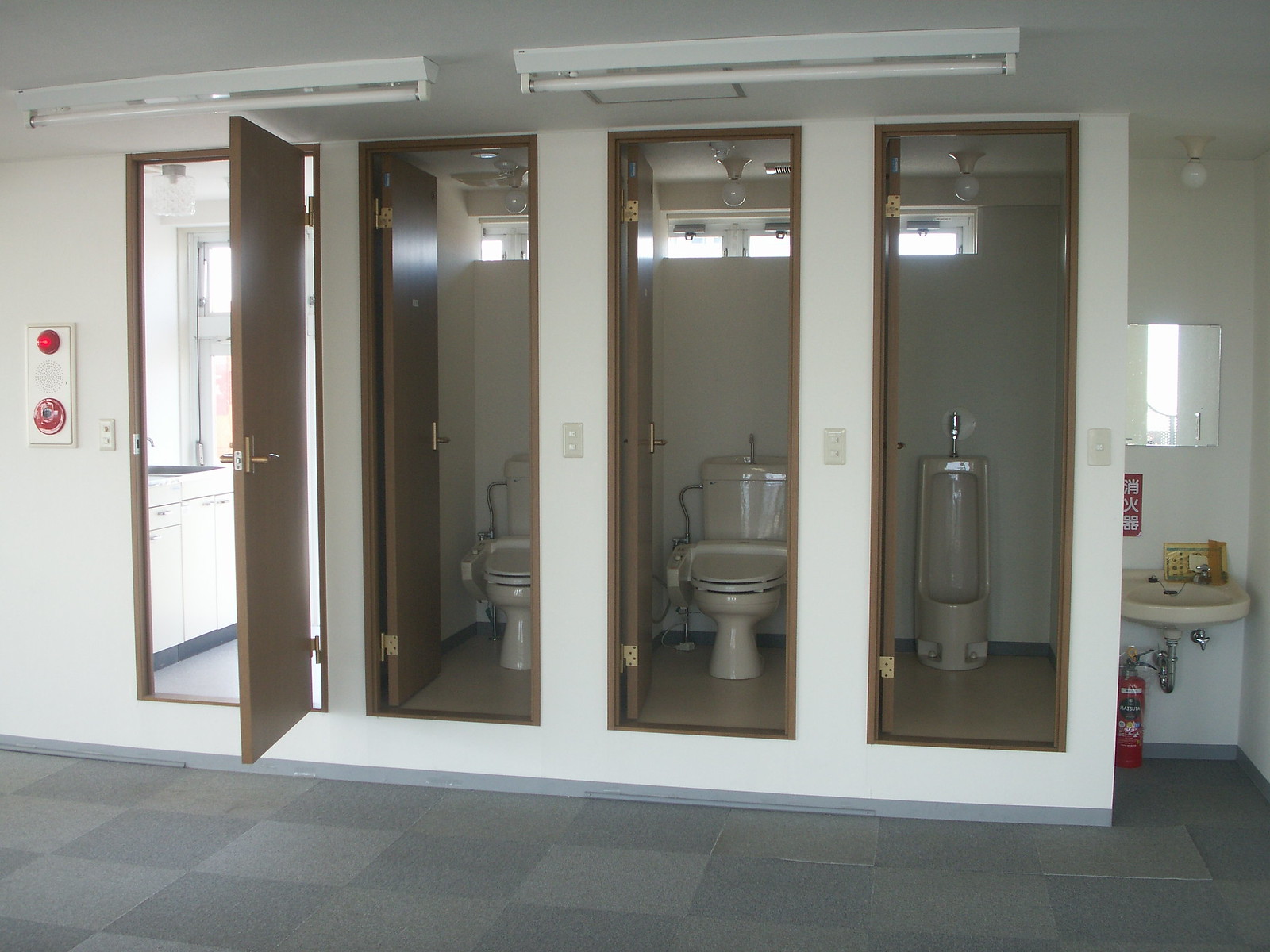This color photograph, taken indoors, captures an immaculately clean bathroom, possibly in an Asian country, featuring a row of four wooden bathroom stalls doors lifted above a tiled gray floor. Each door is brown with small sections of wall between them, all open and facing left. Behind the first door, you see a bathroom sink with a white cabinet and a mirror above it, with a fire extinguisher and a red plaque containing Asian text positioned underneath the sink. The second stall reveals a white toilet with a small window at the top of the wall. The third stall, similarly, houses another white toilet accompanied by a small window at the very top. The fourth stall contains a white urinal with a small window above it as well. The walls are white, and there are two fluorescent lights in the outer portion of the room, in addition to a lamp hanging at the top.